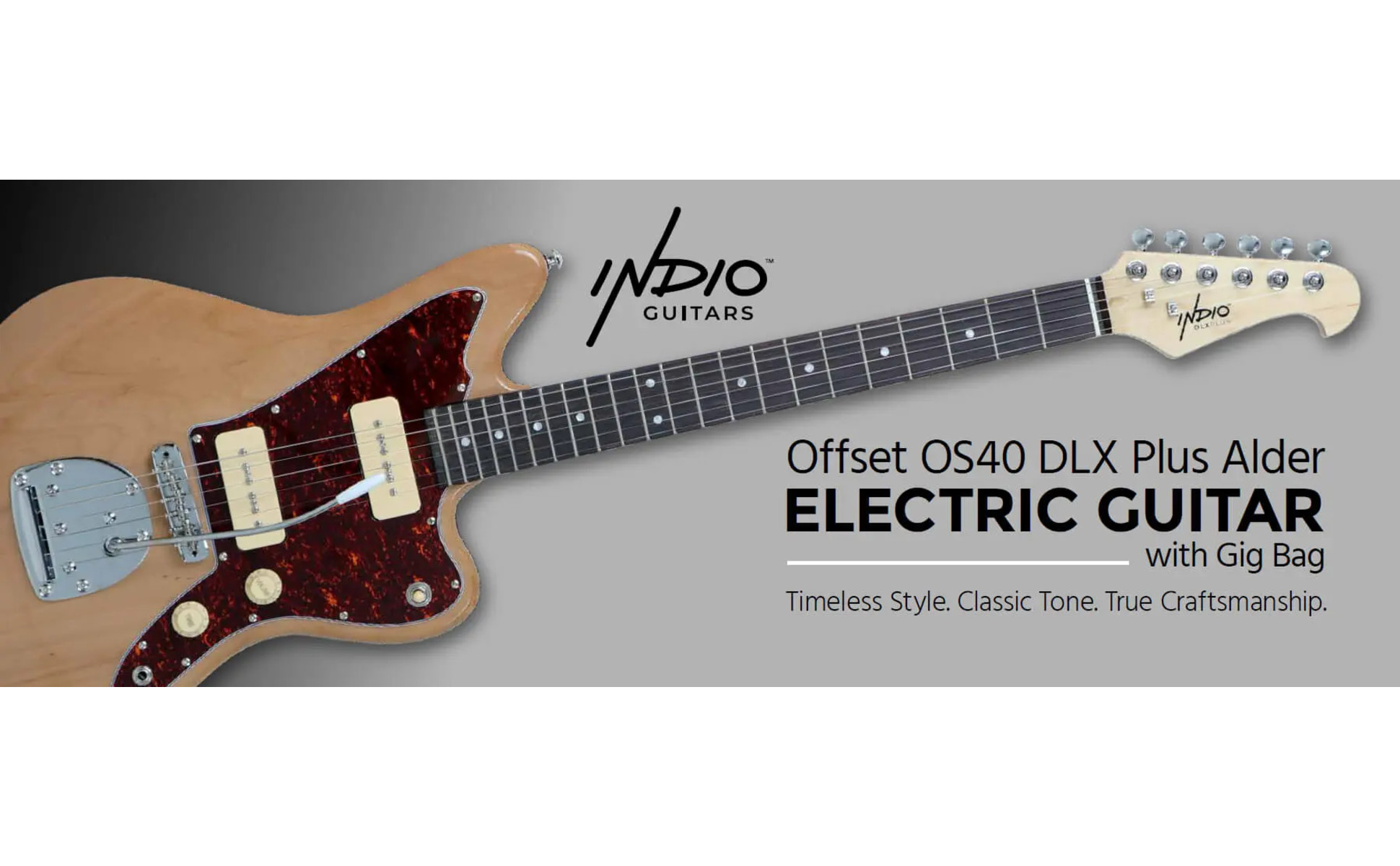The image is a rectangular advertisement for the Indio Guitars Offset OS40DLX Plus Alder Electric Guitar with Gig Bag, featuring timeless style, classic tone, and true craftsmanship. The background transitions from light gray to an ombre darker gray and black in the top left corner. The main focus is the electric guitar, positioned diagonally with its body touching the bottom left corner and its neck extending toward the top right. The guitar has a light brown wood-stained body, complemented by a darker cherry-red, glossy faceplate resembling the material used for guitar picks. The neck is a darker brown, while the headstock is a nearly white lighter wood stain, adorned with silver knobs and the brand name "Indio." The image is wider than it is tall, and in the bottom right corner, the text reads "Offset OS40DLX Plus Alder Electric Guitar with Gig Bag. Timeless style, classic tone, true craftsmanship," separated by a white line. A whammy bar is attached to the guitar, enhancing its classic visual appeal.